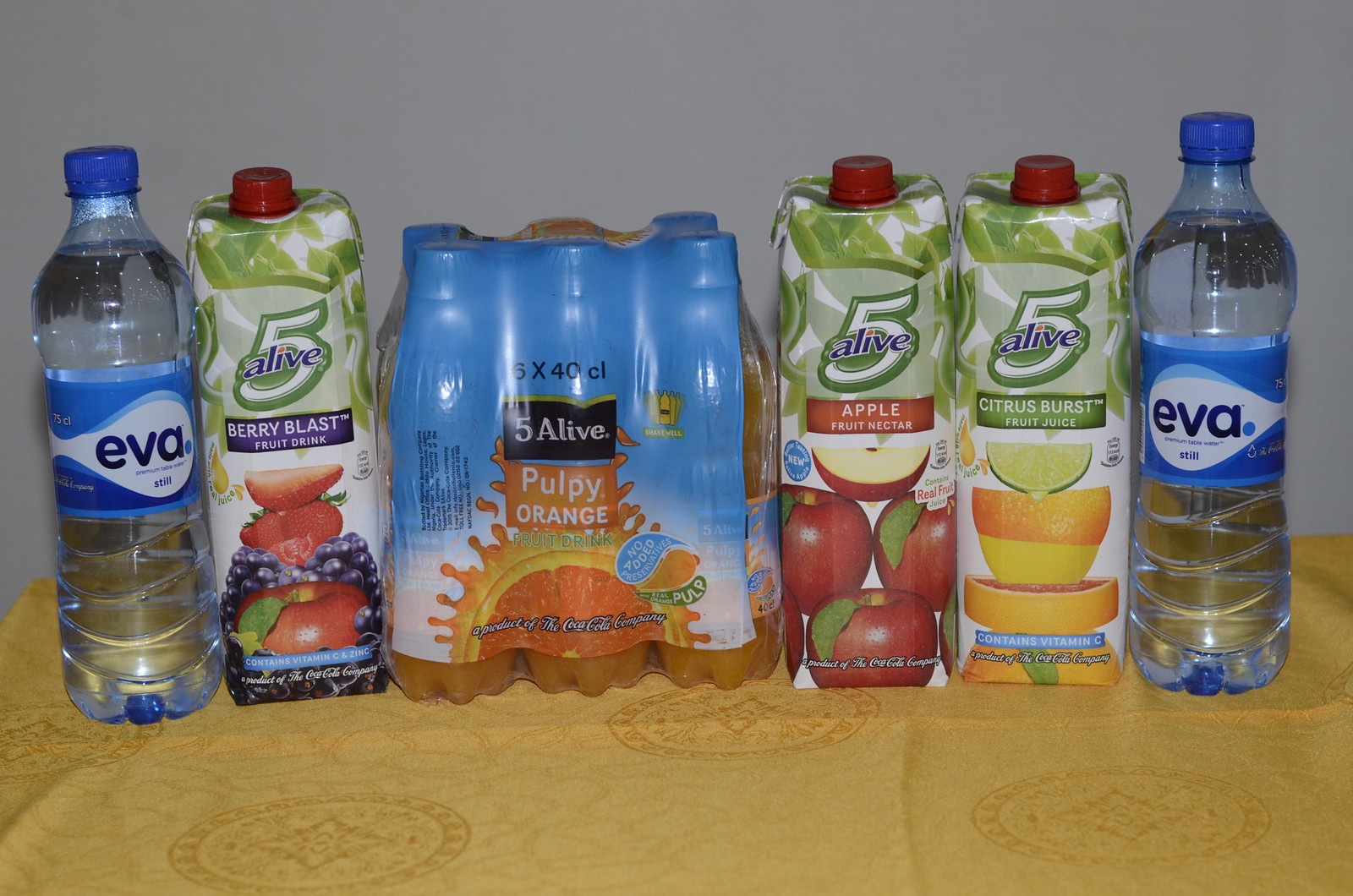This image showcases a neat lineup of various drinks on a yellowish patterned dining room tablecloth, which features noticeable creases from being folded. Positioned from left to right, the arrangement begins with a bottle of EVA water, identifiable by its blue lid and blue logo stating "EVA" with "still" written below. Next to it is a carton of Five Alive Berry Blast fruit drink, followed by a six-pack of Five Alive Pulpy Orange Juice, marked as having no added sugar and containing pulp. Continuing to the right is a carton of Five Alive Apple Fruit Nectar, succeeded by Five Alive Citrus Burst fruit juice. The row concludes with another EVA water bottle. Each beverage stands out with its vibrant packaging, adding a colorful contrast to the yellow tablecloth backdrop.